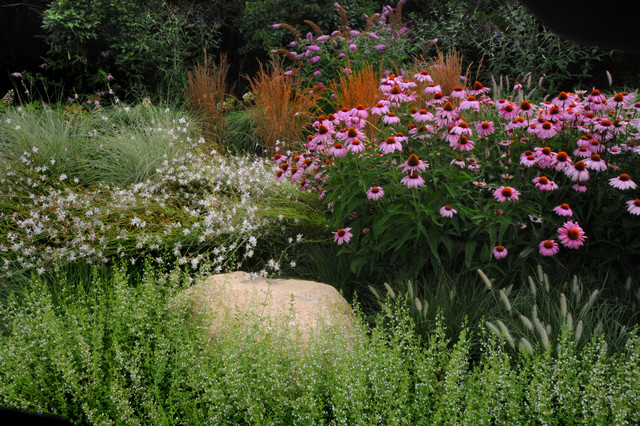This vibrant outdoor photograph, taken in bright daylight, showcases a picturesque scene reminiscent of a public botanical garden or arboretum. The foreground is adorned with lush green ferns and other decorative grasses interspersed with wild oats. A large, tan boulder is prominently positioned slightly off-center to the left, surrounded by an array of shrubs and plants. On the left side of the image, numerous white wildflowers intermingle with tall grass, creating a delicate contrast. Dominating the right side, a dense bush features purple flowers with striking red centers, their long petals adding a vivid splash of color. Nestled between these purple blooms and the shrubs is a plant with long green stems topped with soft, cotton-like white fluff. The background reveals a dense forested area, which casts a darker shade among the trees, enhancing the brightness of the foreground flora and contributing to the image's tranquil, natural ambiance.